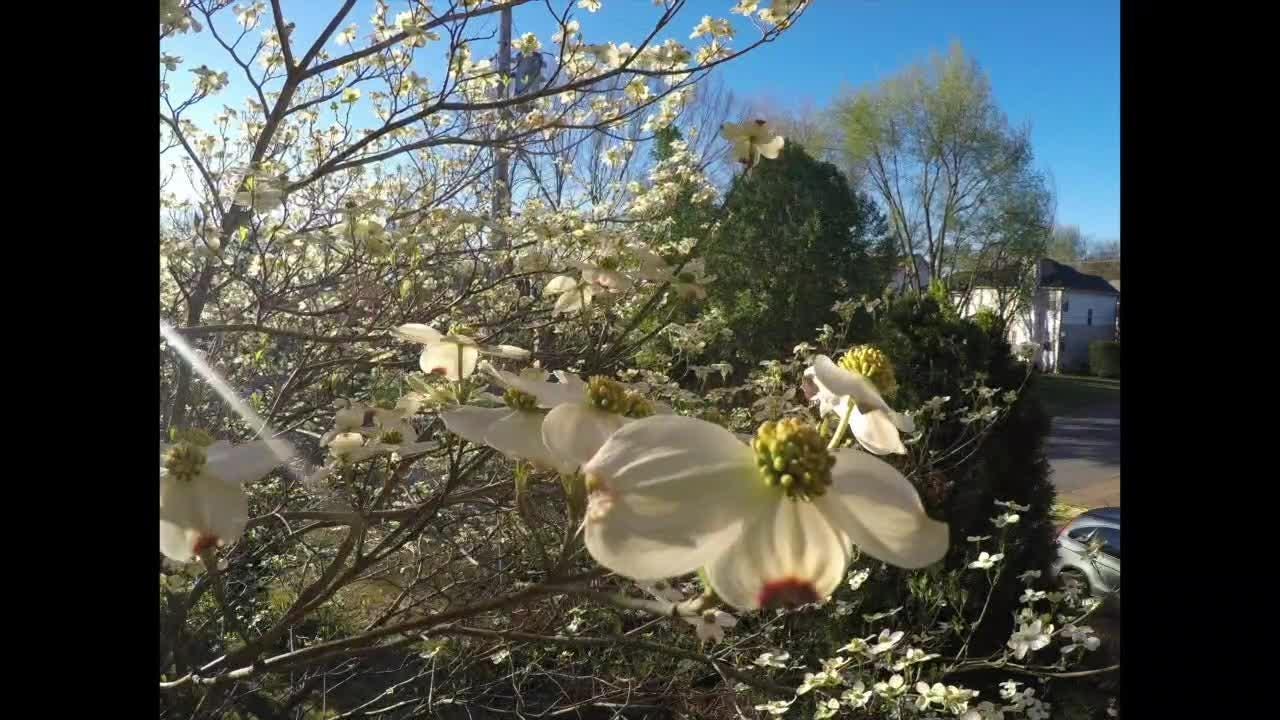The image, possibly from a Ring Video Doorbell or an older camera, shows a close-up view of white blossoms with green centers on tree branches, almost as if seen from the perspective of a pollinating bee. The photo has a fisheye effect and black borders on either side. In the foreground, the branches with delicate white petals and small red divots dominate the scene. To the right, a house stands with a large tree beside it and a car visible in the lower corner near the road. The background features a blue sky, devoid of clouds, and some coniferous trees. A lens flare caused by the sun is visible on the left side, adding to the bright, clear feel of the image.